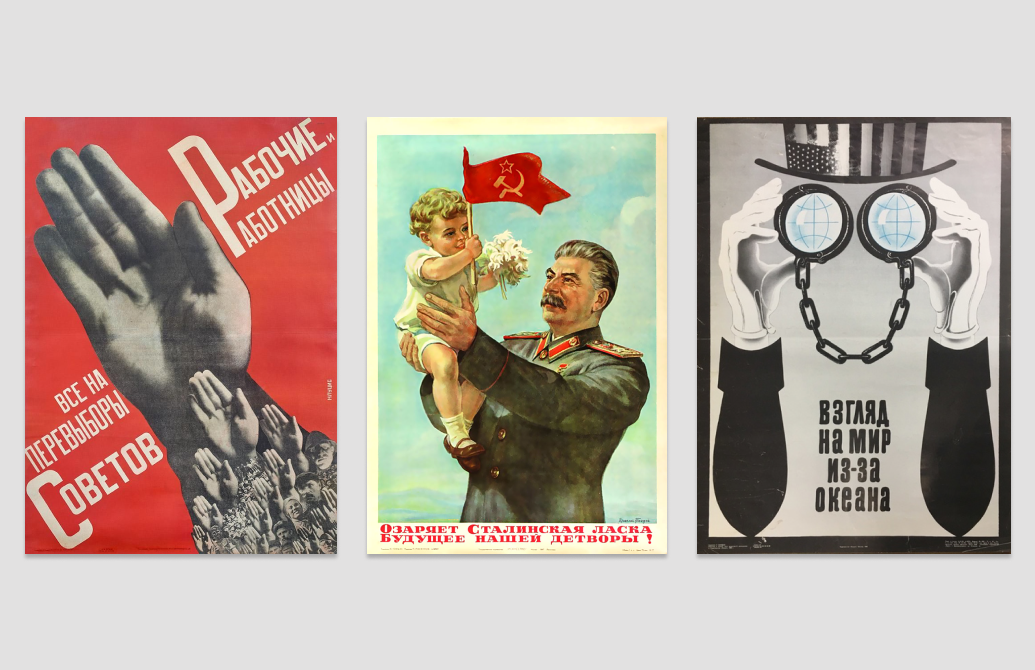This image features a trio of Soviet-era propaganda posters, meticulously arranged side by side from left to right, all set against a light gray background. The leftmost poster presents a striking red backdrop adorned with a large, diagonal hand that is surrounded by several smaller hands beneath it. The poster is emblazoned with white text written in a foreign language, likely conveying a motivational statement from bottom left to upper right.

The central poster showcases a vivid blue background with a detailed drawing of Joseph Stalin holding up a child. The child is proudly gripping a flag of the Soviet Union, which is red with a gold hammer and sickle topped by a gold star. Below this uplifting image, text in Russian, written in red, spans the width of the poster.

The rightmost poster contrasts sharply with its black-and-white drawing featuring two hands holding magnifying glasses in front of an invisible face, giving the impression of eyes. Atop this invisible head is a hat adorned with the USA flag, suggesting a critical view of America. The only color in this poster is the blue tint of the magnifying glasses. Black text, once again in a foreign language, is situated in the middle of the image, against a light gray background, aligning with the overarching motif of propaganda.